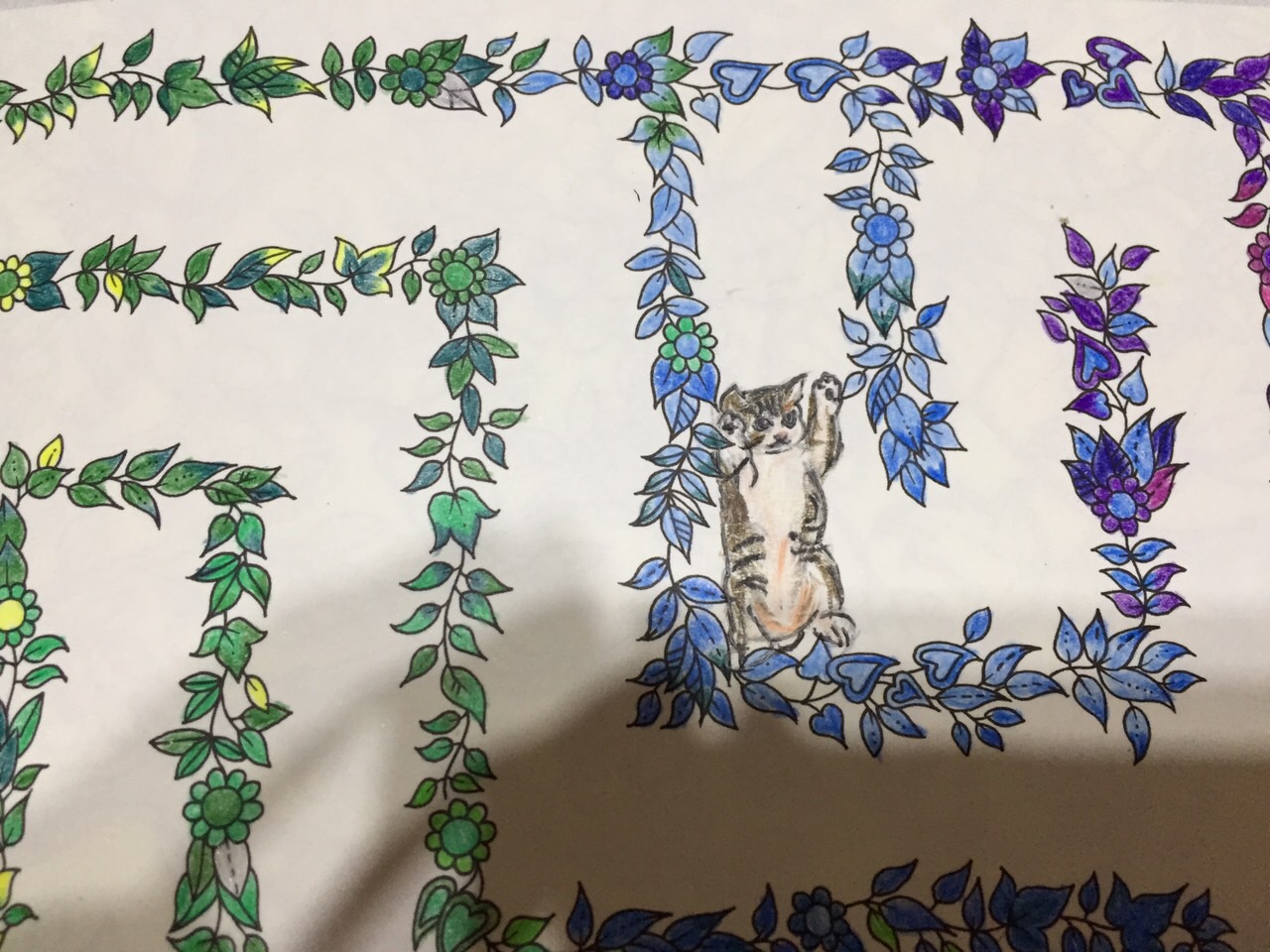The image depicts a realistic photograph of a hand-drawn artwork, meticulously crafted with pencil crayons. At the heart of the illustration, amidst a complex, maze-like structure made up of parallel branches and sharp 90-degree turns, sits a small, gray, and white cat. This cat, drawn predominantly in graphite with subtle lighter tones on its belly, has its paws raised in the air, giving an impression of being stuck in the intricate maze. 

The maze itself is composed of various leaves and flowers, arranged in a straight line across the top edge, with branches extending downwards and weaving through the image. The left side of the maze features foliage in shades of green, yellow, and occasional touches of blue, while the right side shifts predominantly to hues of blue and purple with interspersed red-purple tones, creating a layered, rainbow-like effect. The entire artwork is set against a white or off-white background, with a shadow cast on the bottom right, suggesting the presence of the photographer. 

The artistic composition of the leaves and flowers gives the maze a vibrant yet sophisticated appearance, creating a mesmerizing contrast with the grayscale cat at its center.